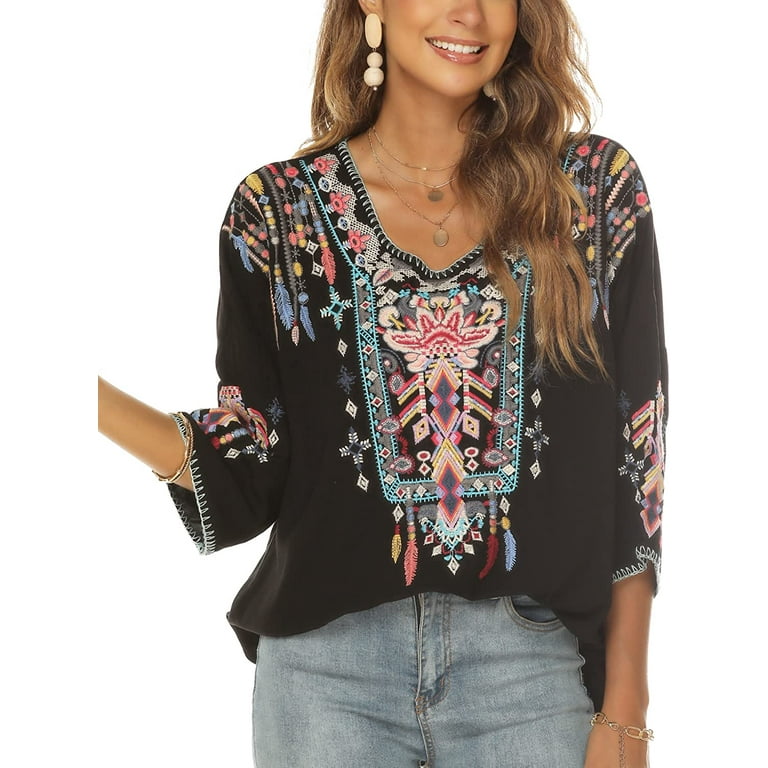This image features a woman standing against a white background, resembling a fashion advertisement likely found on a website or in a catalog. The woman, whose face is partially cut off from nose up with her eyes not visible, has long, light brown wavy hair cascading down. She is adorned with a long, tan-colored earring in one ear, which features an oval shape and two dangling tan balls. She is smiling subtly.

Her outfit consists of a striking black top with long sleeves that extend halfway down her arms. The top is richly embroidered with an intricate, multicolored design incorporating pink flowers outlined in white, feathers, and abstract patterns reminiscent of Native American and Aztec artistry. The elaborate embroidery includes shades of yellow, purple, red, and pink, and has some features that resemble suns or tassels. She pairs this with light-colored denim jeans.

Accessories include a bracelet on each wrist, a few necklaces, and two large pearl-like earrings. The overall styling and white background suggest the image is intended to showcase the outfit in a commercial context, highlighting the details and craftsmanship of the tribal-inspired top along with the complementing light denim jeans.